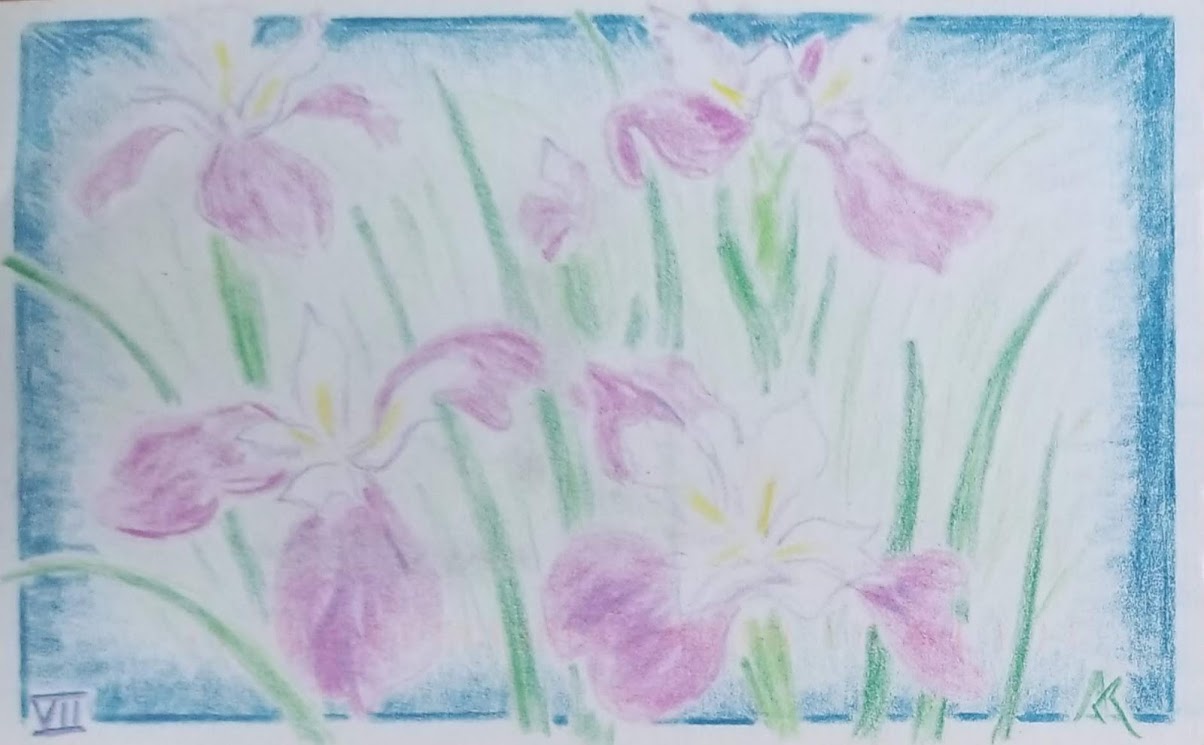This image appears to be a detailed crayon drawing, bordered by a gradient frame transitioning from dark blue to turquoise, creating a striking pattern along the edges. Within this frame, the artwork depicts tall, thin green stalks transitioning from light to dark green, giving them a dimensional look. The drawing showcases four to five vibrant flowers, resembling irises or lilies, characterized by their four petals each. The petals exhibit a gradient from light purple to pink or lavender, with central white highlights and yellow stamens. Some of the green stalks extend beyond the border, enhancing the depth of the image. The lower left corner of the white background features the Roman numeral VII, while the lower right corner bears the artist's initials resembling "MR." The horizontal composition of the piece and the meticulous crayon technique contribute to its captivating and vivid visual appeal.